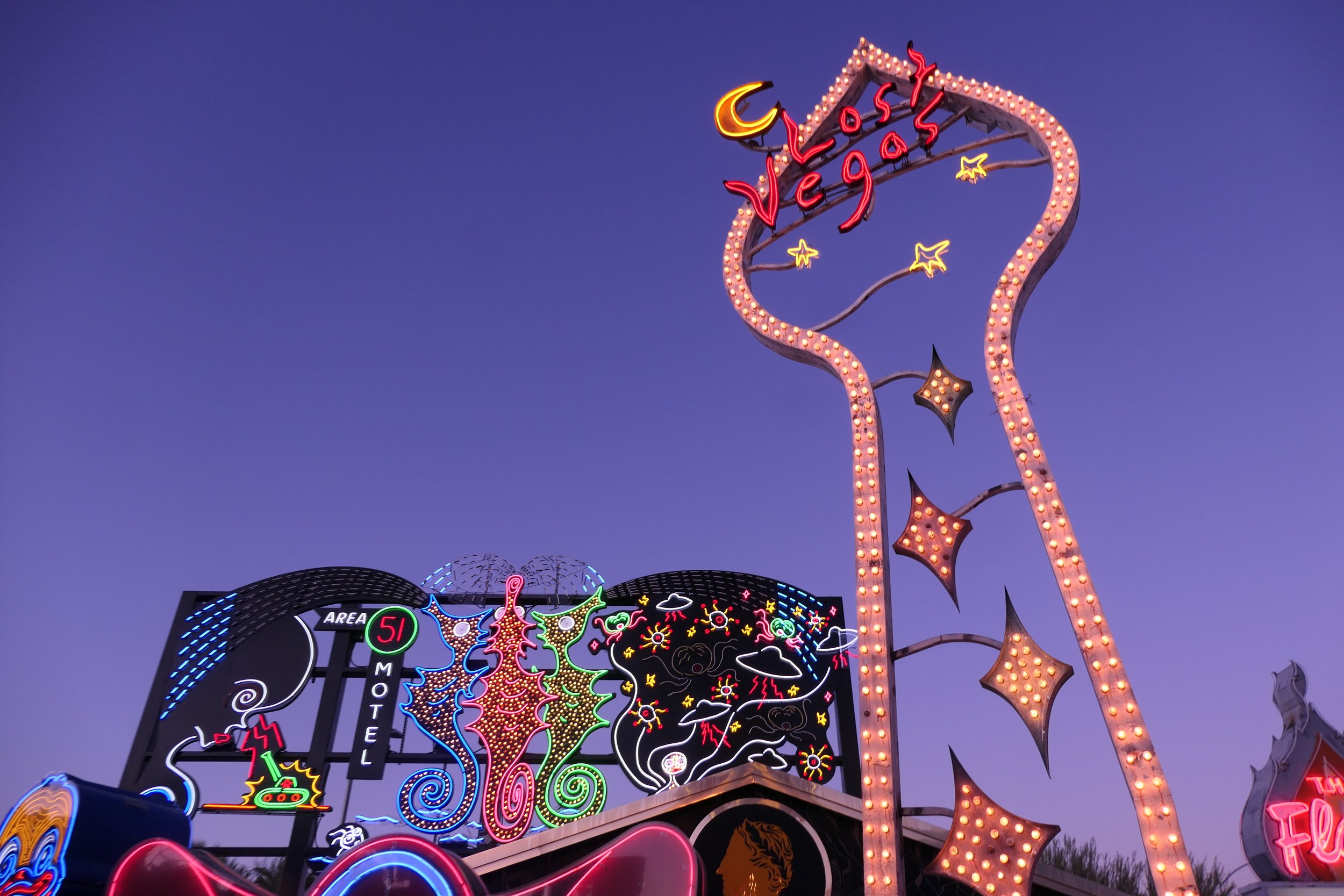In this captivating image, set against a clear, perfectly blue sky with no clouds in sight, we see an array of vibrant, old-school neon signs illuminated by colorful light bulbs. Central in the composition is a tall, pointed structure on the right side, emblazoned with the words "Lost Vegas" in glowing red letters. At the top of this sign, there is a moon-like shape, while below, three bright yellow stars add to the nostalgic charm. Directly beneath "Lost Vegas," a partial view of the letters "FL" suggests additional signage not fully captured in the shot.

Adjacent to this is a roofline of a building adorned with a fascinating collection of signs. Prominently featured is an "Area 51 Motel" sign against a black background, decorated with three striking neon seahorses in blue, pink, and green hues. Adding to the whimsical scene, several lights resembling spaceships float nearby, evoking a playful extraterrestrial theme. To the far left, a hint of a possible lit-up clown figure adds another layer of colorful intrigue, though it's partially obscured from view. This image beautifully blends elements of classic Vegas kitsch with a twilight or dusk setting, creating a mesmerizing and nostalgic visual experience.